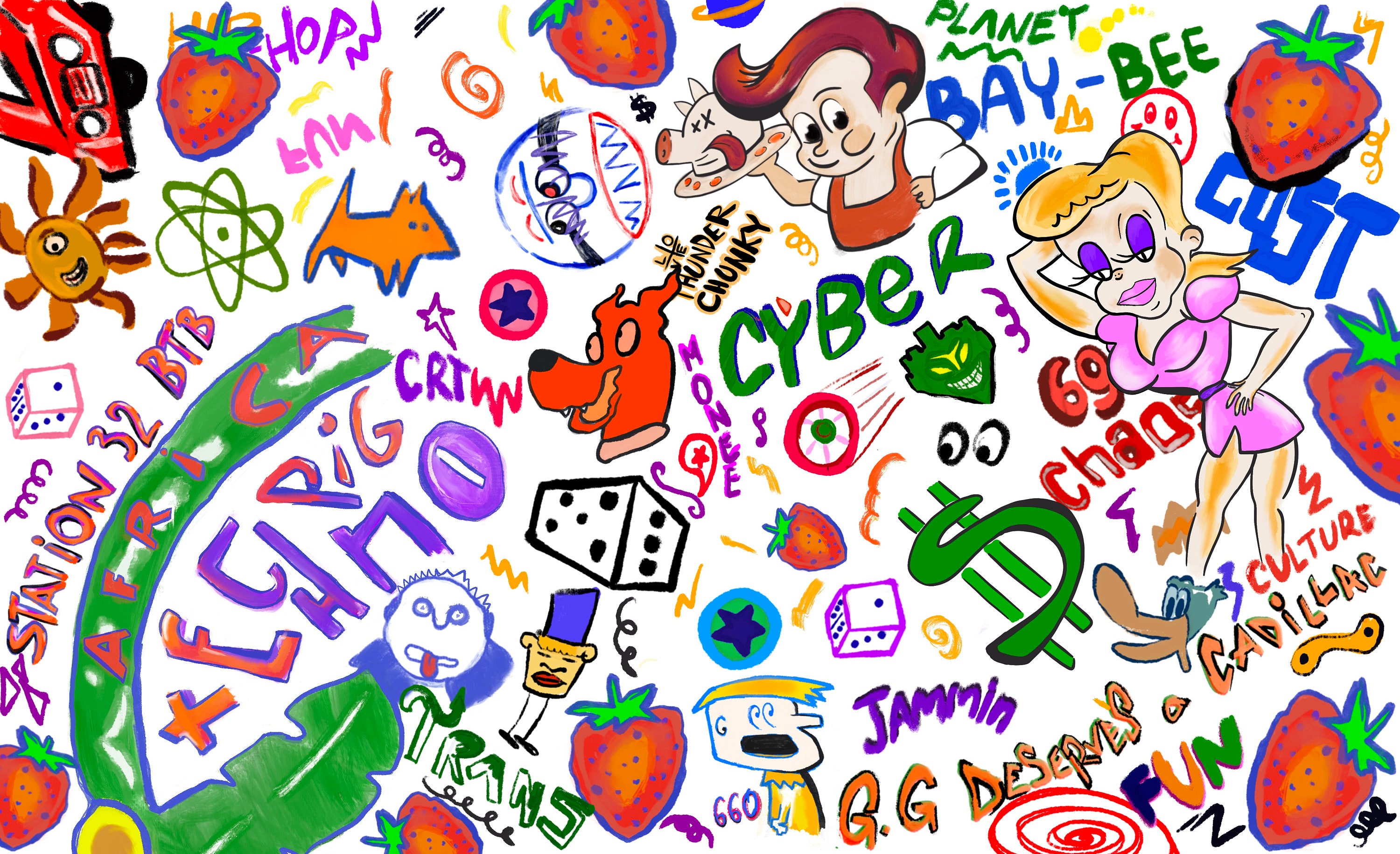The image is a digital, landscape-oriented drawing set on a white background, packed with colorful, chaotic doodles that resemble children's drawings. Among the multitude of elements, notable ones include numerous red strawberries with blue dots and neon green tops, a blonde pinup-style cartoon woman with dark purple eye makeup, dressed in a pink outfit, and a cartoon boy with brown hair wearing an orange apron, holding a plate with a pig's head. Additionally, there's a plethora of text in various colors, reading "Cyber," "Planet," "Baby," "Gust," "Hops," "Station 32," "BTB," "Rig," and "H&O." The imagery is complemented by a variety of symbols such as eyeballs, a green money sign, vibrant shapes, dice, stars, and a sunshine with one eyeball and teeth. Noteworthy mentions include a red swirly design, random characters, and phrases like "Africa" in red on a green stripe and "trans" in green. The entire composition is vibrant and filled with a mix of reds, greens, pinks, purples, making it a visually busy and random scene that would be impossible to detail in full.